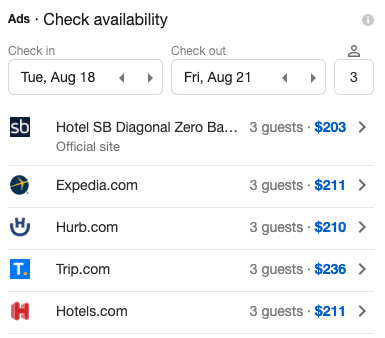In the given screenshot, we see an advertisement detailing accommodation availability and prices for a stay from Tuesday, August 18th to Friday, August 21st. The ad includes pricing options for three guests from various booking platforms. Specifically, the prices are as follows: $203 from Expedia, $211 from Herb.com, $210 from Jerk.com, and $236 from Hotel.com. Each price is displayed in a distinct blue font, while "three guests" is written in a light gray color for emphasis.